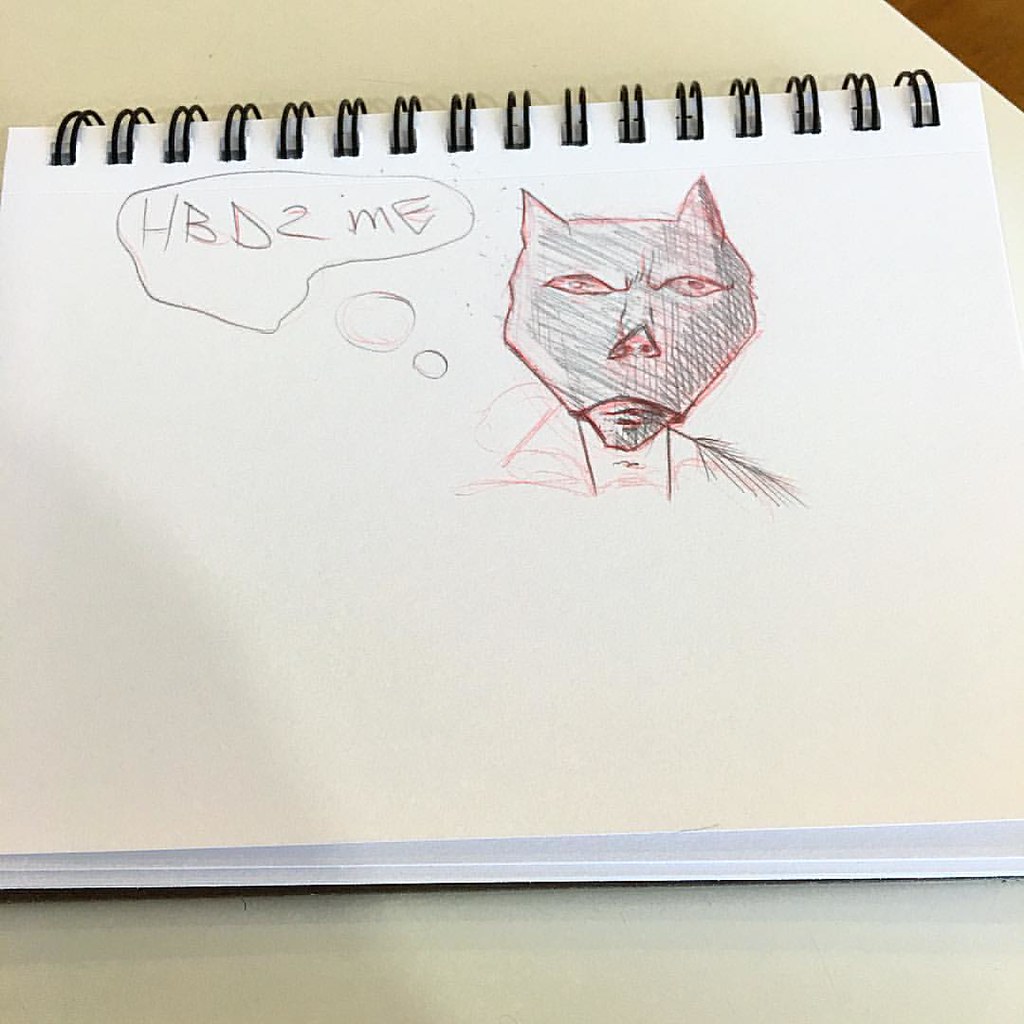Indoor color photograph looking down at a sketch pad set on a white tabletop, captured at a slight angle. The sketch pad, featuring black spirals at the top, has a single detailed drawing on the right side of the page, slightly off-center. This drawing is a cat face with a menacing expression, characterized by a furrowed brow, triangular ears, almond-shaped eyes, and a deep frown. The cat appears to be wearing a jacket. The sketch employs both red outlines and black shading extensively. A thought bubble to the left of the cat's head reads "HBD2ME." The lower eighth of the image reveals the edge of the sketch pad and part of the white tabletop. In the upper right corner, there is an indeterminate brown object. No additional text or elements are present in the photograph.